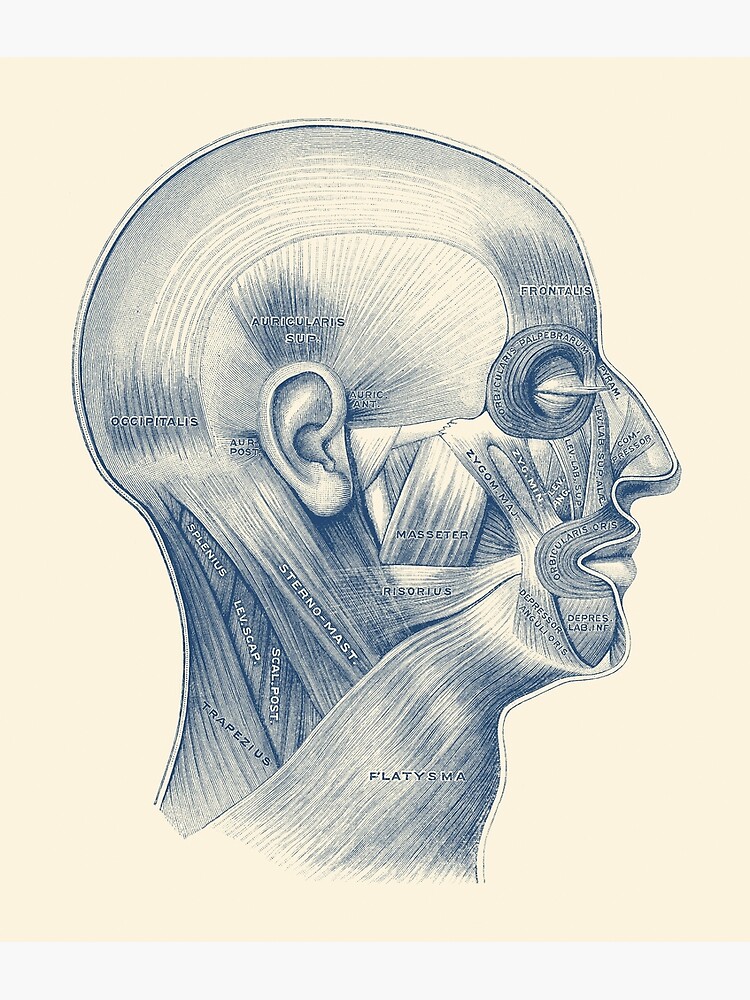The image is a detailed medical artist's rendering of the right side profile of a human head and neck, sketched primarily in pencil with a blue and white color scheme. The background is an ivory or light pink color, making the intricate pencil shading stand out. The drawing meticulously highlights various anatomical features and muscle structures of the face and neck. Labels, primarily in Latin, identify different sections: "frontalis" on the forehead, "auricularis sub" at the center of the head, "occipitalis" at the back, and terms like "splenius," "levator scapulae," "scalp posterior," and "trapezius" along the neck. Additional labels such as "platysma" appear on the front and side of the neck, with smaller inscriptions detailing areas around the nose and eye socket. The precision of the illustration captures both the muscular and skeletal elements, serving as an educational tool for understanding human anatomy.